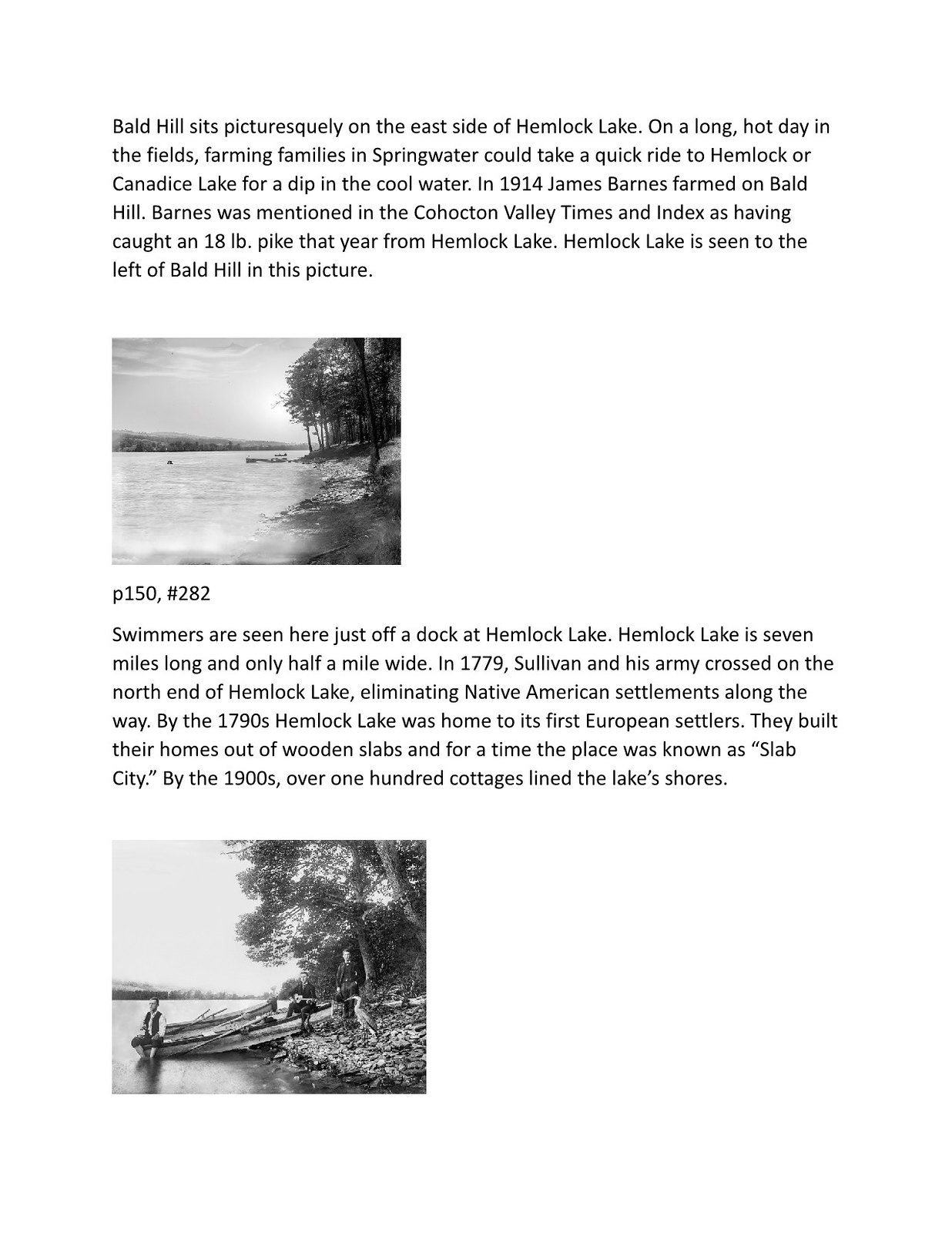The image features a detailed scan or photograph of a book page with a transparent background, highlighting a stark contrast between the white background, black text, and grayscale images. At the top, the primary block of text begins with "Bald Hill sits picturesquely on the east side of Hemlock Lake on a long hot day in the fields." It describes how farming families, during spring water, could make a quick trip to Hemlock or Candace Lake for a refreshing dip. It also references James Barnes, who in 1914, farmed on Bald Hill and caught an 18-pound pike from Hemlock Lake, as reported by the Cohocton Valley Times and Index. To the left of Bald Hill, Hemlock Lake is visible, depicted in a thumbnail image below the text. The caption under this image reads "P150, #282." Another block of text further down explains that swimmers are seen just off a dock at Hemlock Lake, and details the lake's dimensions of seven miles in length and half a mile in width. Historically, in 1779, Sullivan's armies crossed the north end of Hemlock Lake, eliminating Native American settlements. By the 1790s, European settlers established 'Slab City' with homes built from wooden slabs along the lake's shores, and by the 1900s, over 100 cottages had been constructed. This is illustrated by another thumbnail showing the lake's shore, swimmers, and a boat. The layout is informative, intended to educate readers about the local history and picturesque aspects of Hemlock Lake and Bald Hill.